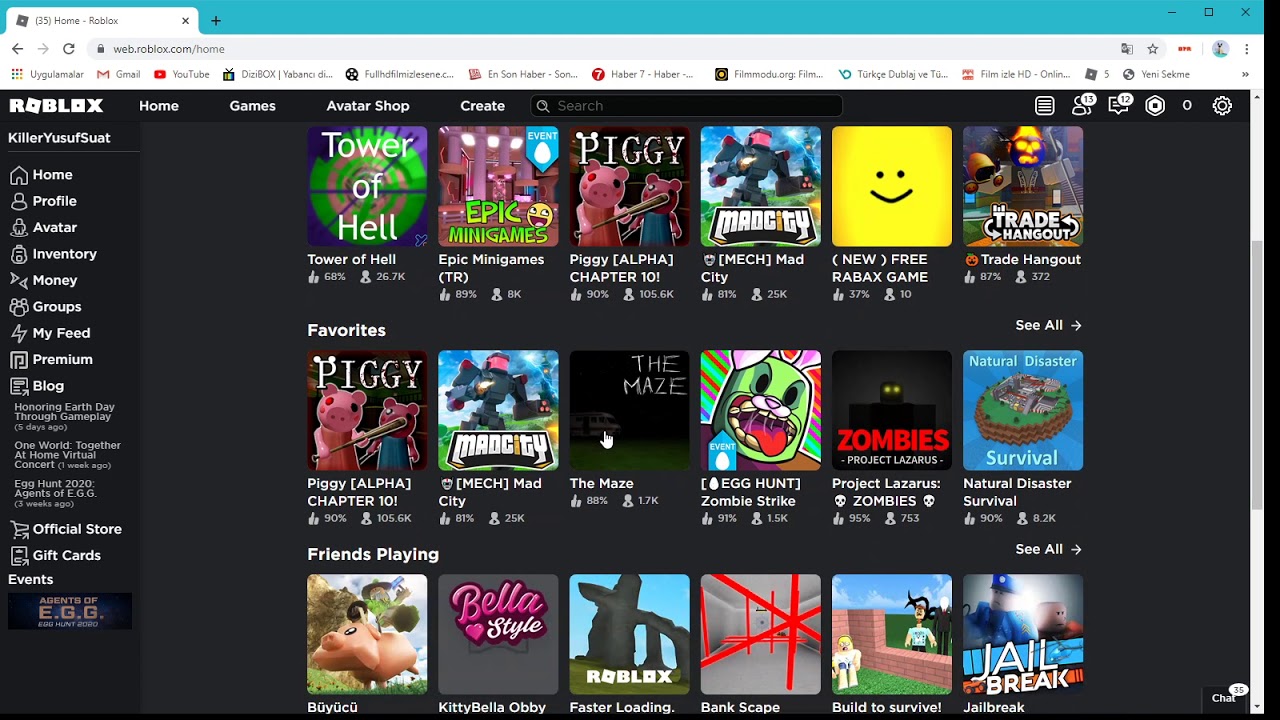This screenshot captures a detailed view of a Roblox-themed website interface, predominantly featuring white text on a black background. The top of the screenshot displays the browser tab with the title "35 Home Roblox," while the main section has a turquoise-colored upper bar containing close buttons on the right. Below this, a typical web browser interface is visible, including back and forward icons and the URL web.roblox.com.

A row of bookmarks is located beneath the address bar, featuring links to Gmail, YouTube, and several other truncated bookmarks. The left sidebar prominently shows the Roblox logo in white, followed by navigation options such as Home, Games, Avatar, Shop, Create, and a search bar. Various icons are also present on the right, displaying notifications such as 13 over a person icon, 12 over a message icon, and a settings gear icon.

Further down the left column under the Roblox heading, there are additional navigation options listed as: killer, you so sue it, Home, Profile, Avatar, Inventory, Money, Groups, My Feed, Premium, and Blog—all displayed with white icons.

The main body of the screenshot highlights recent blog entries, with titles like "Honoring Earth Day through Gameplay" (posted five days ago), "One World Together at Home Virtual Concert" (posted one week ago), and "Egg Hunt 2020" (posted five weeks ago). Below these blog entries, there appears to be a gallery divided into three rows with six squares each, showcasing various content.

The visible top row highlights games such as "Tower of Hell," "Epic Minigames," "Piggy," "Mech," "New Free Roblox Game," and "Trade Hangout," each represented by unique cartoon icons. The second row features favorites like "Piggy," "Mech," "The Maze," "Egg Hunt," "Project Lazarus," and "Natural Disaster."

The bottom section, partially visible, seems to belong to a "Friends Playing" gallery, containing five squares with cartoon icons, though the text underneath is not entirely legible.